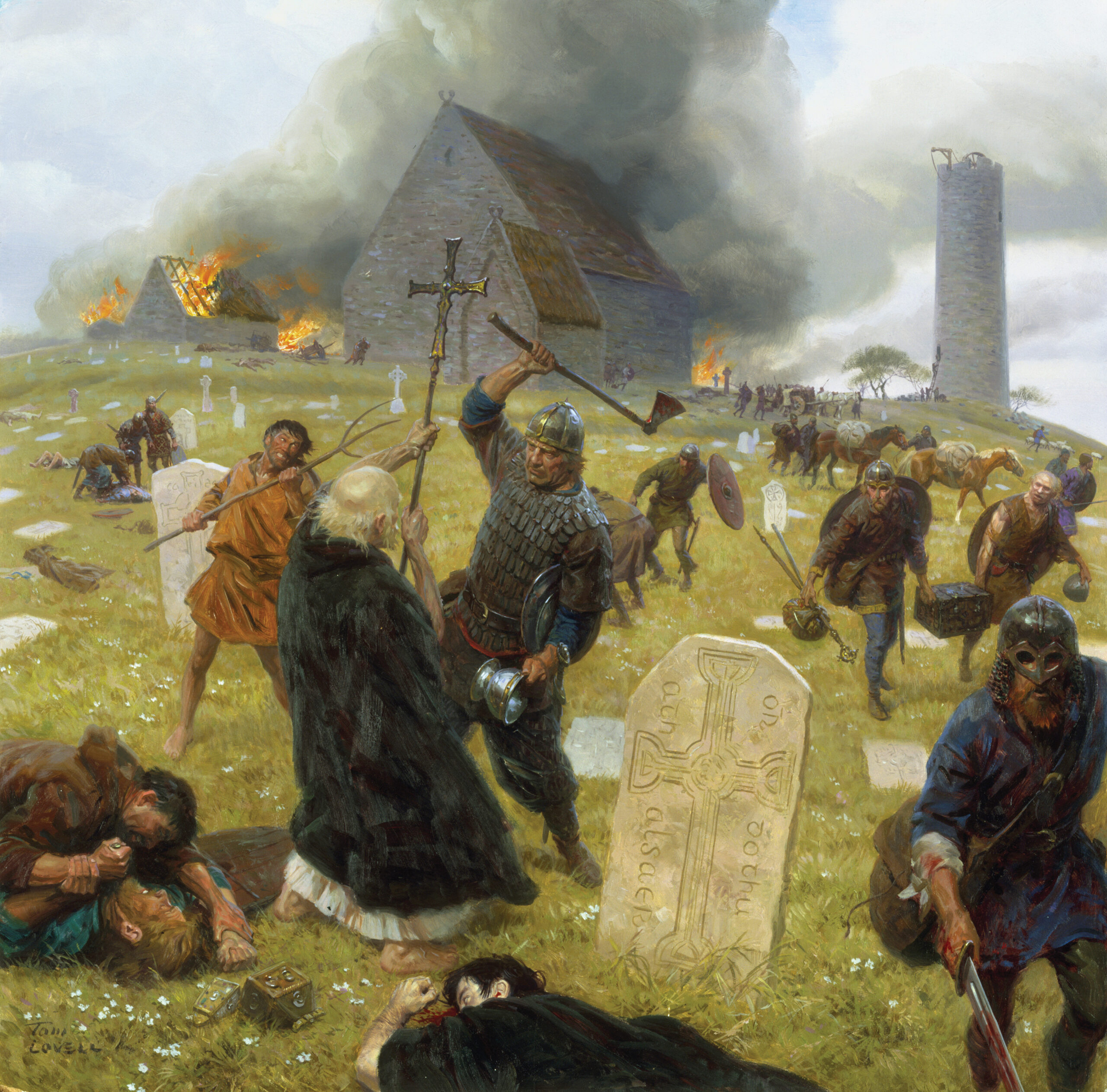The image portrays a vivid and chaotic scene of a Viking raid on a Christian village set on a hillside cemetery. Tombstones are scattered throughout the foreground, where a slain man in a black cape lies sprawled on the ground, while next to him, two men are engaged in a fierce struggle. One combatant, dressed in animal skins, appears to be overpowering his opponent. 

At the center of the turmoil, an older priest, distinguished by his brown hair and black coat, desperately holds aloft a cross mounted on a long rod, his body leaning backward in a defensive posture. Looming over the priest, a Viking warrior, identifiable by his metal helmet, prepares to deliver a lethal blow with his raised axe. Near this intense confrontation, another figure with a rake participates in the melee, though his allegiance remains unclear.

In the background, the village is engulfed in flames. A church and several houses are ablaze, with dark smoke billowing menacingly into the sky. One house, only starting to burn, contrasts starkly with two others that are already half-consumed by fire. Amidst the havoc, Viking raiders can be seen carrying away treasure, including a silver bowl and a treasure box, likely plundered from the village. Another Viking, wielding a blood-encrusted sword, strides away from the dead man in the foreground.

This harrowing depiction captures the brutal violence of a medieval Viking raid, a grim testament to the relentless ravages of war in a European countryside setting from the Middle Ages.